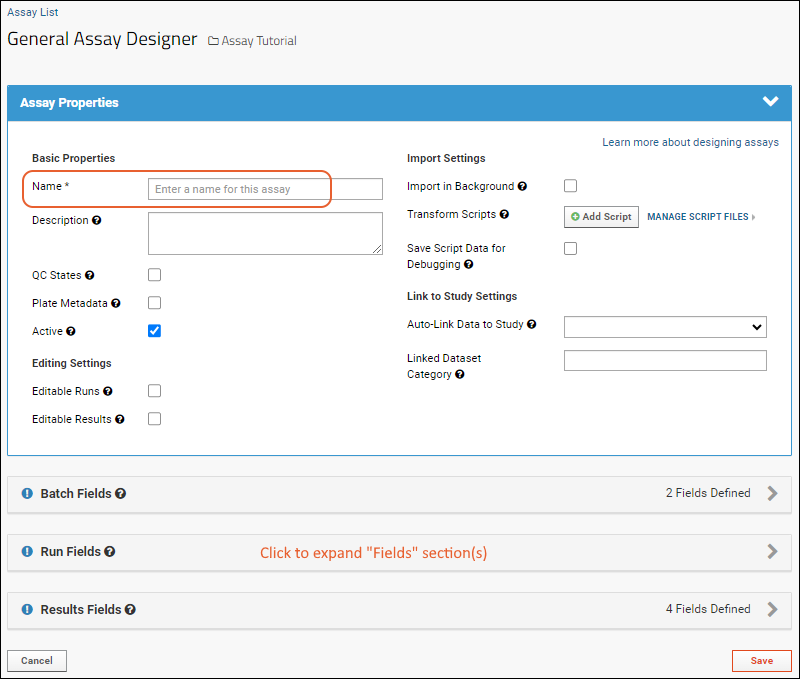Here's a detailed and cleaned-up caption for the provided image:

---

**Caption:**

Screenshot of the General Assay Designer interface, specifically showing the assay list and relevant design options. At the top, a large blue header is prominently displayed with the title "General Assay Designer" followed by "Assay Tutorial" and "Assay Properties." Towards the right side of the header, a down arrow icon is opened, revealing an expanded field.

The expanded field includes various properties and settings for the assay. The "Basic Properties" section instructs the user to enter a name for the assay, which is highlighted with an orange marking. Below this, an area labeled “Description” is provided for additional details. The “QC states” section, along with "Plate Metadata," are displayed with checkboxes, where only the "Active" checkbox is checked, while others remain blank.

Further down, the "Editing Setting" section includes options such as "Editable runs" and "Editable results," both of which are unchecked. In the "Import Settings" section, the “Import background” option is also unchecked. The "Transform Scripts" subsection offers options to "Add script" and "Manage script filters," with an informational link to "Learn more about designing assays" highlighted in blue. The option to "Save script data for debugging" is unchecked.

The "Link to Study Settings" section includes an “Auto-link data in the study” dropdown menu which is not activated, as well as a field for "Link data set category" which remains blank.

Towards the bottom, several sections with expandable fields are displayed, namely "Batch fields," "Run fields," and "Results fields." “Run fields” has an orange marker prompting users to click to expand the fields section. Two specific areas within "Run fields" indicate "2 fields to find" and "4 fields to find," respectively.

Finally, at the bottom-left corner, there is a "Cancel" button, and at the bottom-right corner, an orange "Save" button is present, ready for user interactions.

---

This caption provides a thorough description of the interface, detailing the layout and functionality available within this specific section of the General Assay Designer tool.